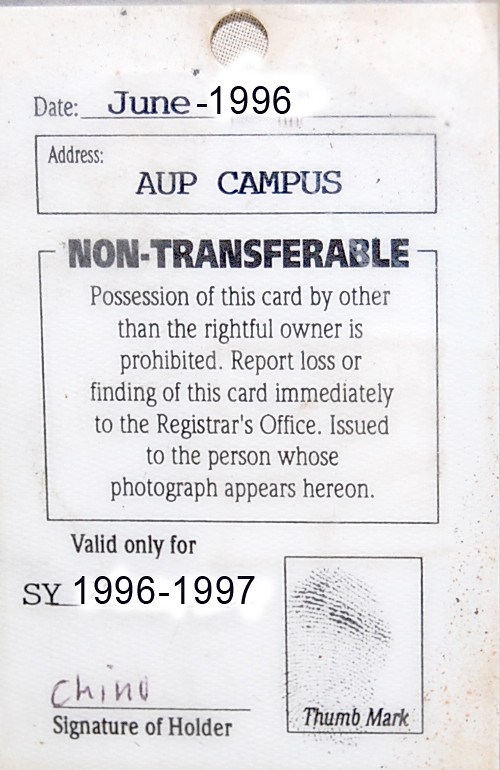The image depicts a detailed scan of an identification card from June 1996. The top of the card has a circle cut out, suggesting it was designed to be hung, perhaps on a strap. The date, "June 1996," appears prominently at the top, seemingly edited post-scan. Below this, a bordered rectangle contains the capitalized text "ADDRESS: AUP CAMPUS." The card features a bold, black text stating "NON-TRANSFERABLE," followed by the admonition "Possession of this card by other than the rightful owner is prohibited. Report loss or finding of this card immediately to the registrar's office. Issued to the person whose photograph appears hereon." It also mentions its validity for the school year, "S.Y. 1996 to 1997," which appears to have been edited as well. Towards the bottom, the card has a handwritten signature, "CHINO," next to which the cardholder's thumbprint is visible, indicating a focus on secure identification. The card shows signs of wear, including dirt marks and a hole at the top, suggesting frequent handling.